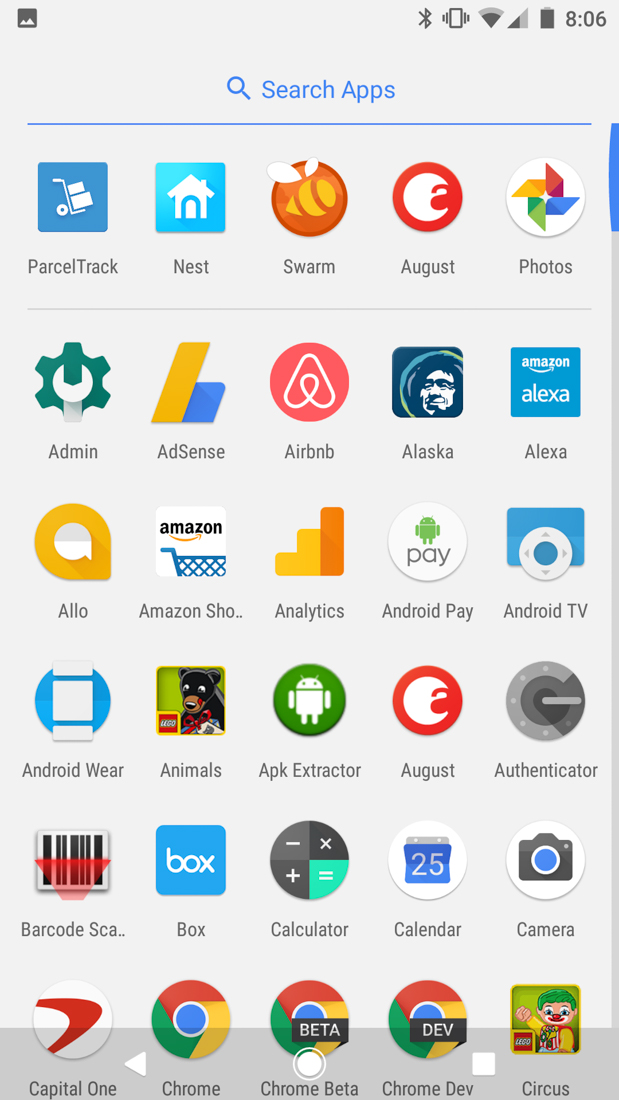This image is a detailed cell phone screenshot, vertically oriented, with a height approximately twice its width. 

### Image Description:
- **Top Section:**
  - **Right Corner**: Indicators for wireless signal, cellular signal, and a fully charged battery.
  - **Time Display**: "8:06" is shown at the top right corner.
  
- **Central Section:**
  - **Search Bar**: Centered at the top is a magnifying glass icon followed by the text "Search apps" in blue.
  - **Blue Bar**: Sits directly beneath the search bar.

- **Main Layout:**
  - **Background**: Gray overall.
  - **App Grid**: Features a 5-column by 6-row layout of app icons, totaling 30 icons.

### Icons Listed (in order):
1. Parcel Track
2. Nest
3. Swarm
4. August
5. Photos
6. Admin
7. AdSense
8. Airbnb
9. Alaska
10. Alexa
11. Allo
12. Amazon
13. Sho
14. Analytics
15. Android Pay
16. Android TV
17. Android Wear
18. Animals
19. APK Extractor
20. August
21. Authenticator
22. Barcode Scanner
23. Box
24. Calculator
25. Calendar
26. Camera
27. Capital One
28. Chrome
29. Chrome Beta
30. Com Developer
31. Circus